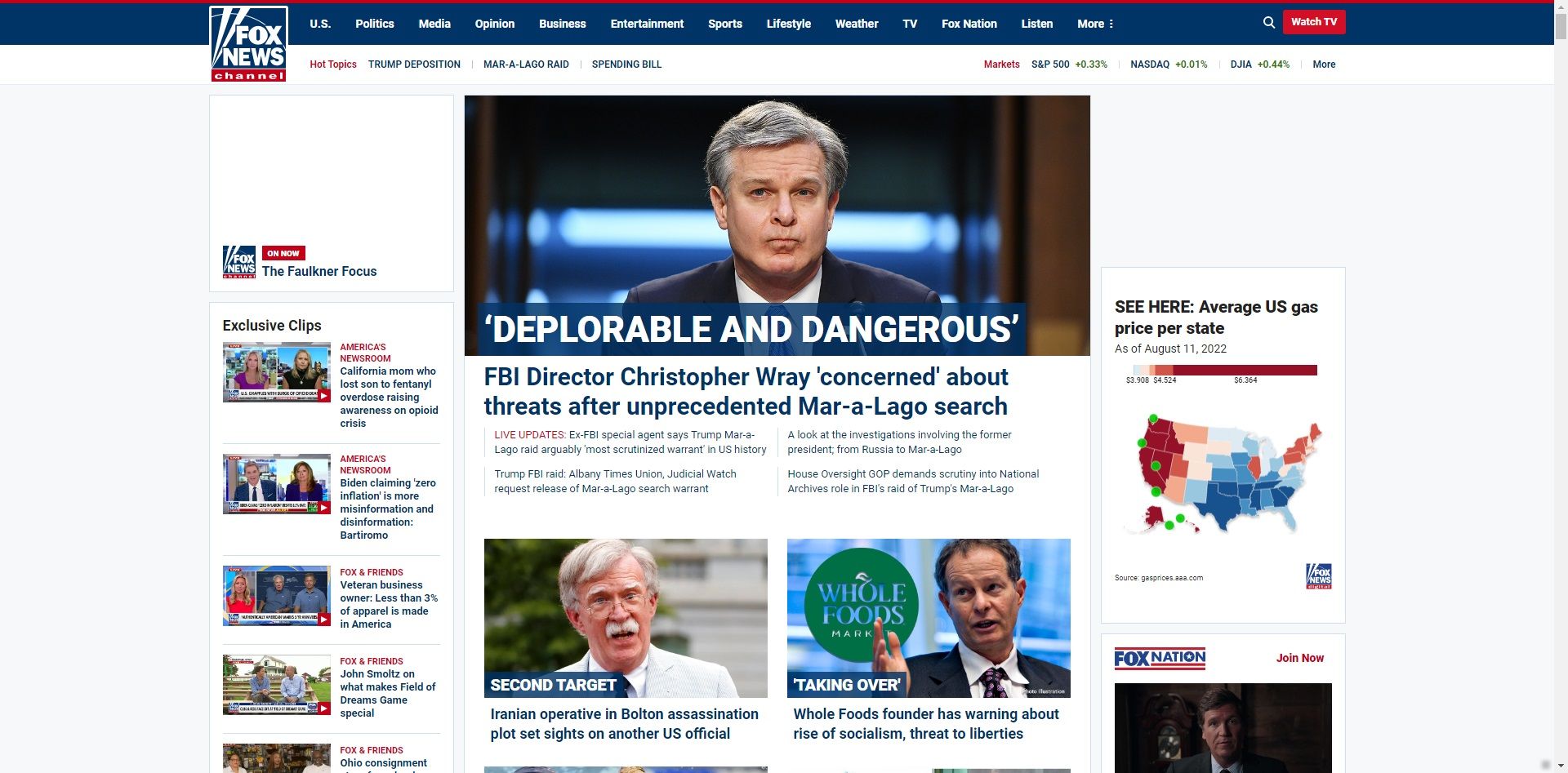The image depicts a webpage from the Fox News Channel. At the top left corner, the Fox News Channel logo is prominently displayed. Below the logo are navigation links categorized under US, Politics, Media, Opinion, Business, Entertainment, Sports, Lifestyle, Weather, CV, Fox Nation, Listen, and More. Featured content includes exclusive clips from "America's Newsroom" and several headlines. One headline highlights a story about a California mother raising awareness on the opioid crisis after losing her son to a fentanyl overdose. Another headline emphasizes FBI Director Christopher Wray's concerns about threats following an unprecedented illegal search. Additionally, it mentions an Iranian operative involved in an assassination plot targeting a second US official, and a warning from the Whole Foods founder about the rise of socialism and its threats to liberties.